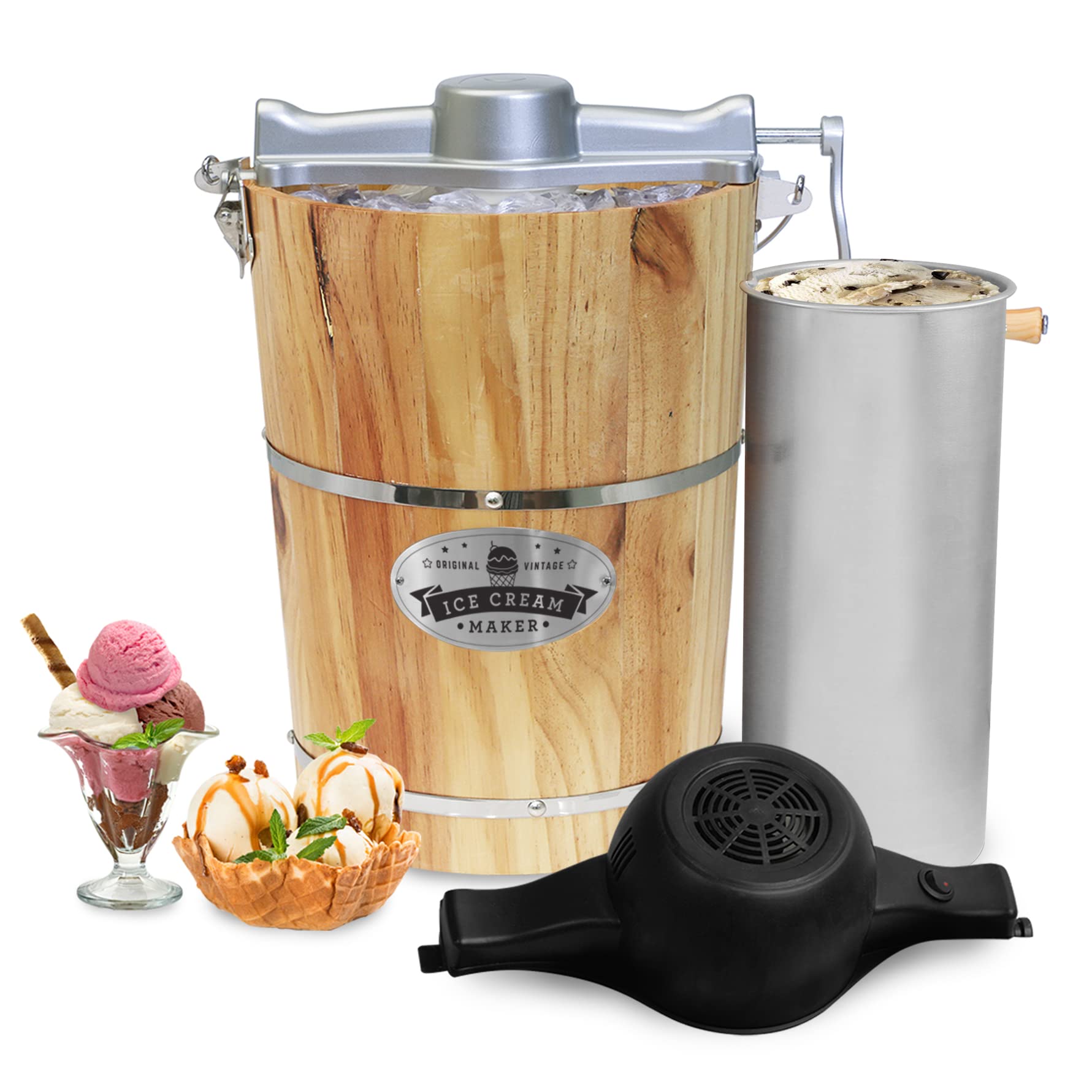This is an image of a vintage-style ice cream maker, displayed on an all-white background. The centerpiece is an old-fashioned wooden bucket with visible vertical grain, secured by multiple stainless steel bands. A silver label on the front reads "Original Vintage Ice Cream Maker." On top, there's an aluminum-colored section with a manual crank handle, depicted in the process of churning ice cream. Inside the bucket, some ice is visible, reinforcing the rustic, hands-on nature of the product.

To the right of the wooden bucket stands a tall silver cylinder, presumably the container where the ice cream is made. It appears to be filled with ice cream, possibly vanilla with chocolate chips or an Oreo-like mix. In front of the cylinder lies a black electrical motor with a fan vent and an on/off switch, offering a modern alternative to traditional hand-cranking.

In the bottom right corner of the image, there's a close-up of a golden-brown waffle bowl filled with vanilla ice cream, caramel drizzle, nuts, and a green mint leaf garnish. Directly to the left lies another ice cream treat in a classic glass sundae cup, showcasing scoops of vanilla, strawberry, and chocolate ice cream, topped with a vanilla stick or biscotti with chocolate stripes, and a mint leaf. These ice cream treats serve to illustrate the delicious end product made by the ice cream maker.